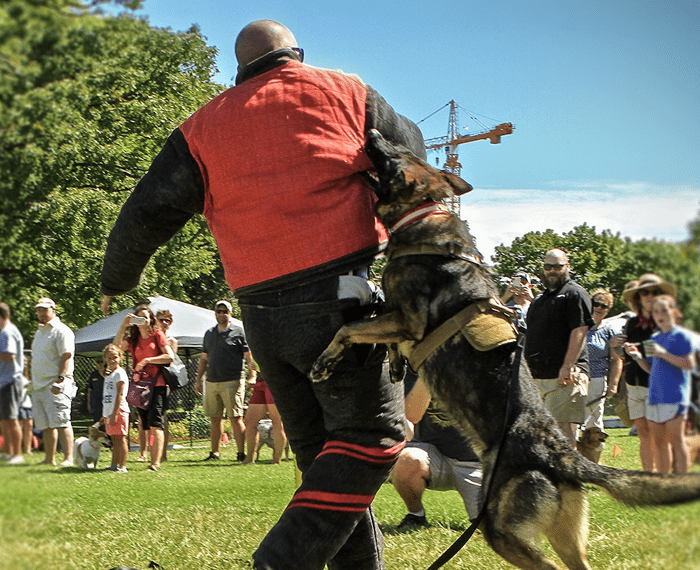The photograph captures a dynamic dog training demonstration in a sunlit park with green grass and surrounding trees. Front and center, a bald man wearing glasses and protective, padded clothing—red and black jacket with matching black trousers featuring red stripes—is being bitten on the arm by a black and brown German Shepherd. The dog, which is equipped with a belt around its face and a military-style halter, is leaping up at the man. A crowd of spectators, a mix of adults and children with some accompanied by their pets, looks on with a mix of smiles and shock. A utility pole stands in the background, blending into the vibrant landscape with blue skies and white clouds.